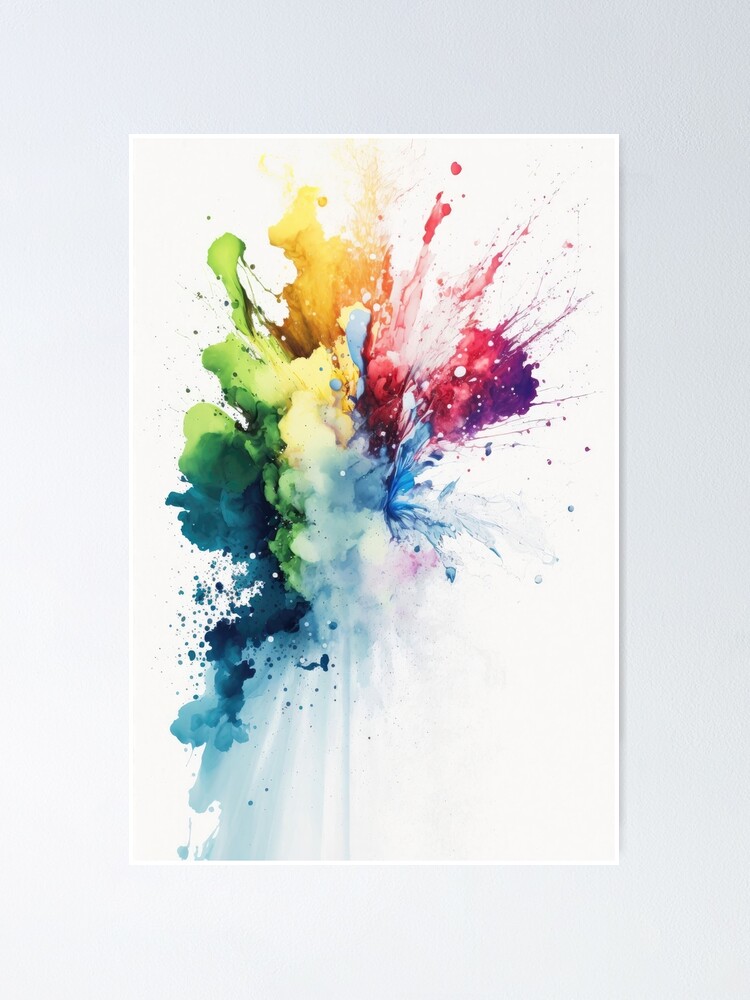This full-color photograph captures a vertically rectangular piece of abstract wall art mounted against a very light blue, almost grayish wall. The artwork itself is also vertically oriented and features a white canvas with an intricate explosion of vibrant paint colors. The outer edges of the art are framed by a light gray border that appears slightly washed out on the lower left side, possibly illuminated by an artificial light source.

The central motif of the painting resembles a vase with paint splotches representing flowers. At the bottom of the canvas, white grooves suggest the vase's structure. Bursting from this base, the painting features an array of vibrant paint splotches and streaks, arranged in a manner that gives the impression of an explosive outward motion. These splotches include dark purple, red, varying shades of orange, yellow, multiple shades of green, different blues, and hints of brown.

On the right, a striking red splotch drips upward, while an orange splotch occupies a central position. Below the orange, a yellow patch and, to the upper left and left, green smudges add complexity. The lower left features bluish-gray hues. Each color appears not just in isolated splatters but also as dots and streaks radiating outward, creating a dynamic and chaotic visual effect. This artistic explosion of colors turns the white canvas into a vivid spectacle of abstract art.